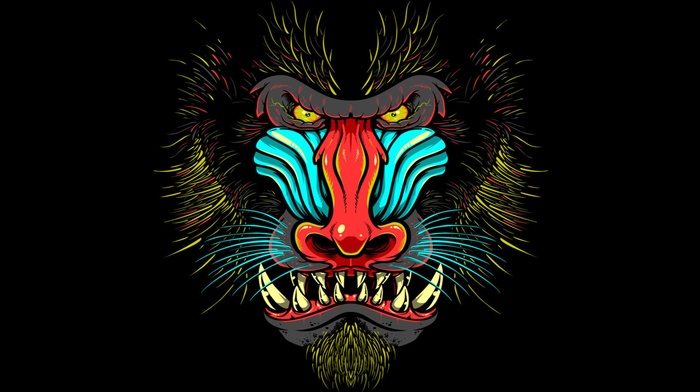This image showcases a vividly menacing cartoon depiction of an ape or gorilla set against a solid black rectangular background. The central focus is the dramatic and highly expressive face of the creature, which exudes an eerie and threatening aura. The ape's face is a mosaic of striking colors; it has piercing yellow eyes surrounded by gray shadows, enhancing its fearsome appearance. The cheekbones are highlighted in turquoise, while the nose and the area around it blaze with a fiery red, complete with wide nostrils. The mouth is agape in a fierce growl, revealing an array of sharp, glimmering white teeth that contribute to its ferocious expression. 

Further adding to the menacing look, the chin is a dusky gray, with greenish-black hair sprouting from its bottom. This hair, which also protrudes from the sides of the face and above the eyes, is an unsettling blend of greenish-black interspersed with striking hues of purple, pink, and occasional specks of red. Completing the intimidating visage are the bright patches of yellow goatee fur. Despite the abstract and animated style, the image conveys a powerful sense of anger and readiness to attack, as if the creature is poised to defend itself or lash out at anyone who dares to confront it.